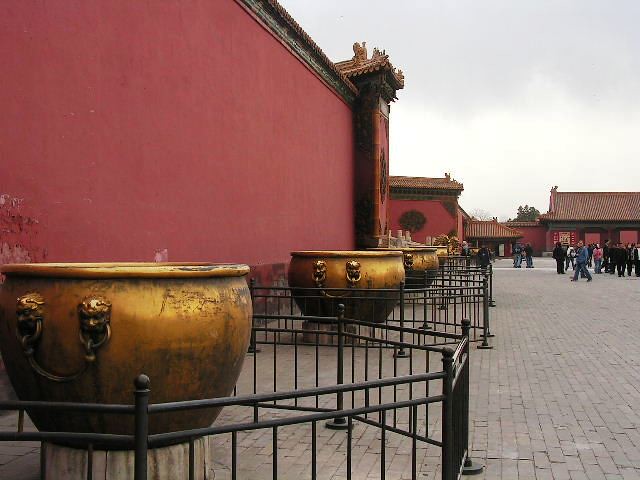This photograph captures an ornate Asian temple complex, possibly in China or Japan, with several distinct architectural and decorative features. Dominating the left side of the image is a towering, crimson wall that stretches from the far left to over halfway through the frame. The wall is intricately detailed at the top with green and gold ornamentation. Prominent gold statues are set at the corner of the wall, adding to its grandeur. 

Adjacent to the wall, there are several large bronze or brassy gold cauldrons, each adorned with creature-head designs, possibly lions, and circular handles connecting at their faces. These cauldrons are surrounded by waist-high, hexagonal black wrought-iron railings, providing protection and adding to the aesthetic appeal. The cauldrons appear weathered, with noticeable black and brown streaks. 

On the right side of the photograph, further in the distance, there are more buildings with strikingly similar architectural styles, featuring crimson walls, detailed green tops, and tan, gold-ornate roofs that curve outwards. A small crowd can be seen in the distance under a gray, cloudy sky, enhancing the serene yet grand atmosphere of the temple complex. The ground surrounding the temples consists of dark-colored bricks, blending harmoniously with the overall color palette of the scene.